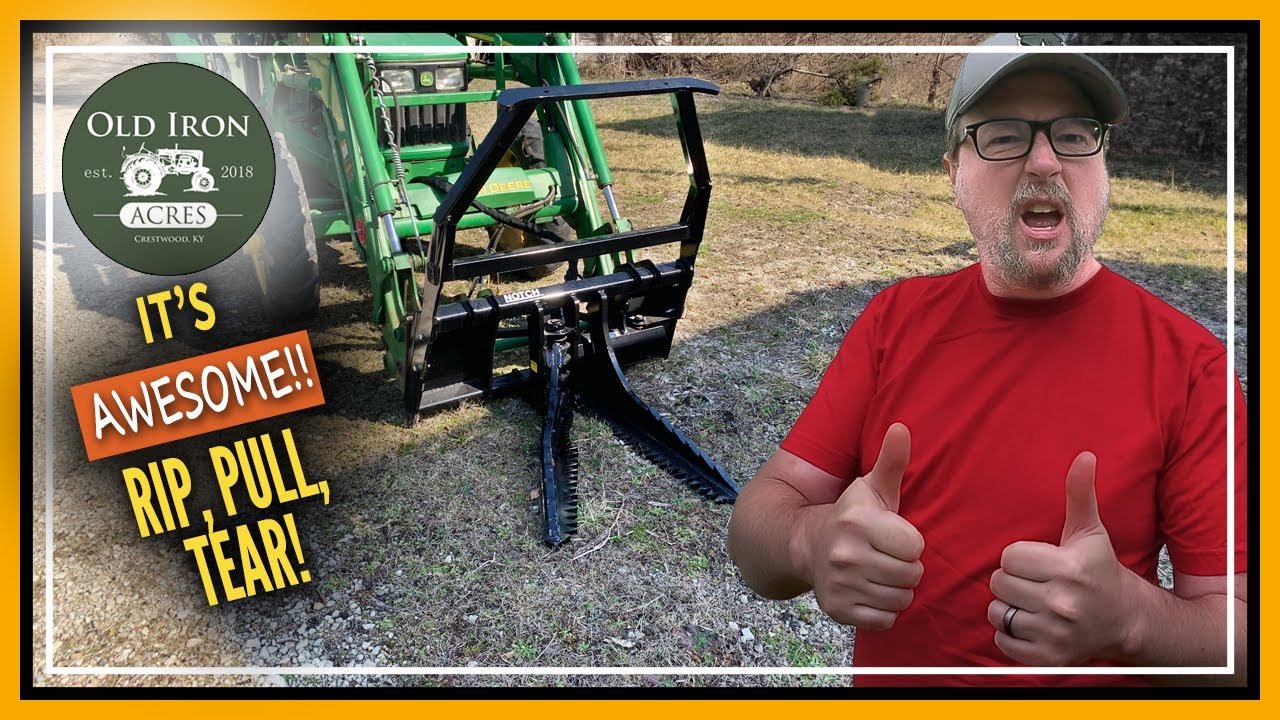This detailed advertisement for Old Iron Acres in Crestwood, Kentucky features a vividly depicted outdoor scene. The photo showcases a fierce-looking piece of green farm machinery on a somewhat unkempt lawn, bordered by brush and forest. The machinery has large wheels and a black, two-pronged attachment at the front, resembling a plow or clippers. Dominating the right side of the image, a man in a red shirt, black glasses, and a white baseball cap strikes a thumbs-up pose. He sports a blonde goatee and has his mouth open as if exclaiming "yeah." The left side of the image includes a circular emblem reading "Old Iron Acres" and text that says "It's awesome. Rip, pull, tear" in yellow and white fonts with an orange rectangular background behind the word 'awesome.' The overall composition is framed by yellow, black, and white borders, creating a striking and dynamic advertisement.